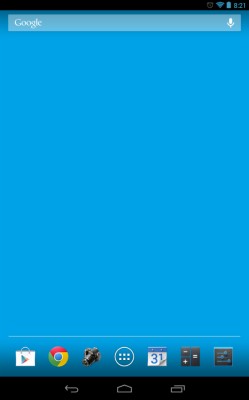The image is a detailed screenshot of a smartphone showcasing various elements of its user interface. At the very top is a slender black border. On the upper right corner, there is the time displayed in blue as "8:21," adjacent to the battery icon, which indicates a full charge. To the left of the battery icon, a full Wi-Fi signal is visible, followed by a gray alarm clock icon.

Below these icons, the screen transitions into a deep blue color that dominates most of the display. At the top of this deep blue section, a lighter blue strip spans nearly the entire width from left to right. On the left side of this lighter blue strip, the word "Google" is written in white, while on the far right, there is a microphone icon.

The majority of the deep blue section remains empty until about two inches from the bottom, where a thin blue line stretches almost completely across the screen. Directly below this line are three icons arranged in a blue circle with a white border, featuring three horizontal dots.

Further down, there is a row of app icons. From left to right, they are:
1. Google Play Store
2. Google Chrome
3. Camera
4. A central circle icon
5. Calendar
6. Calculator
7. A unique black square icon displaying blue lines and circles.

To the left of these icons, there is an arrow icon that points right, then up, and back to the left, forming a circular route. Adjacent to this, towards the right side, are gray outlines of the home and multitasking icons. The home icon is a simple outline of a house, while the square multitasking icon has a gray line extending down and to the right, with another gray line crossing over.